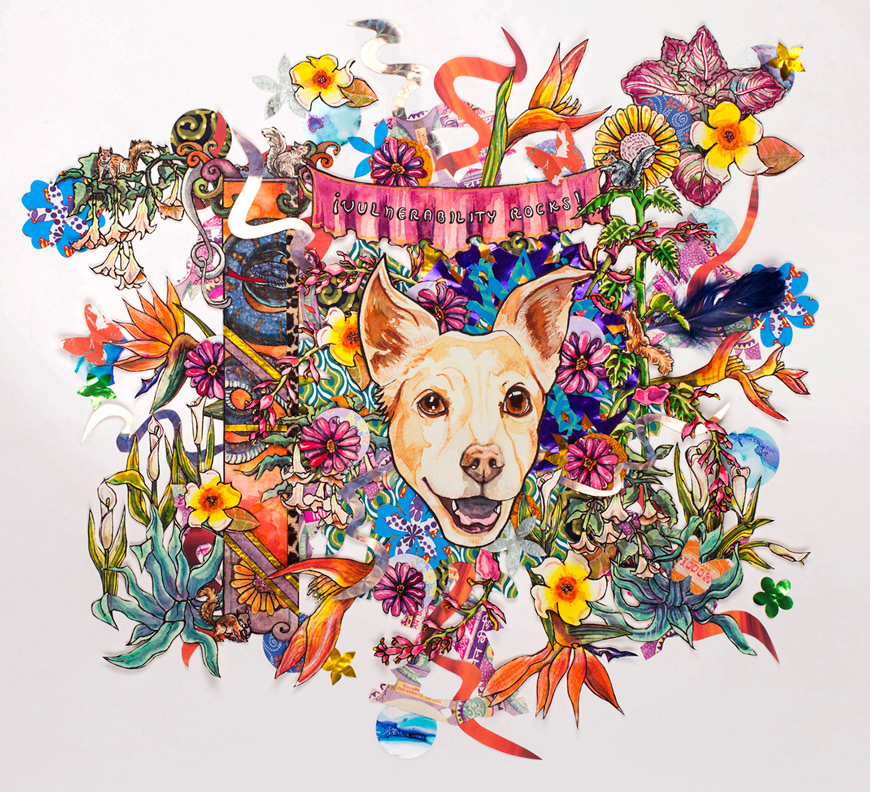This vibrant and eye-catching animated image features the head of a blonde, pointy-eared dog surrounded by an array of multicolored flowers. A ribbon banner, positioned above the dog, reads "Vulnerability Rocks." The flowers encircling the dog are in various hues, including yellow, pink, blue, and orange, with additional details like orange leaves, blue vines, and green elements. The artwork, resembling a collage, is a highly detailed and colorful creation, with additional features like a pillar off to the left, all contributing to its rich, artistic feel.